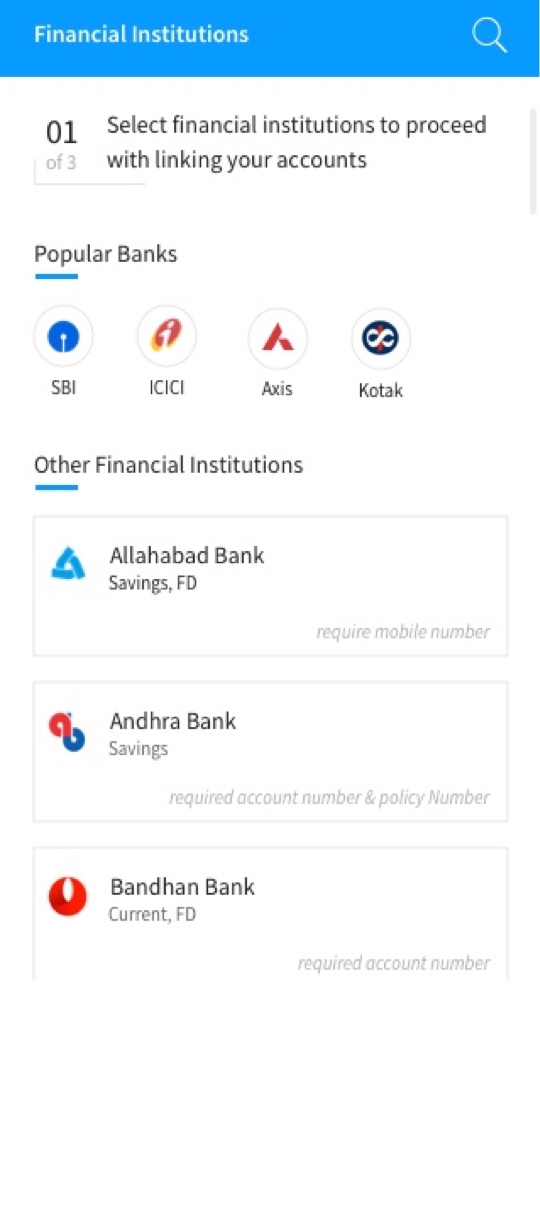The image features a user interface on a white background with a blue header titled "Financial Institutions." Below the header, a white magnifying glass icon is visible, accompanied by the text "0 of 3 selected: Select financial institutions to proceed with linking your accounts."

A section labeled "Popular Banks" is underlined in blue and lists the following banks:
1. SBI
2. ICICI
3. AXIS
4. COTAC

Another section, labeled "Other Financial Institutions" and also underlined in blue, presents three rectangular fields for additional financial institutions:
1. Alhabad (spelled A-L-A-H-A-B-A-D), offering Savings and FD accounts that require a mobile number.
2. Andra Bank (spelled A-N-D-H-R-A), providing Savings accounts that need both an account number and a policy number.
3. Bandhan Bank (spelled B-A-N-D-H-A-N), featuring Current and FD accounts that require an account number.

A gray scroll bar is located on the right side at the top of the interface for navigation.